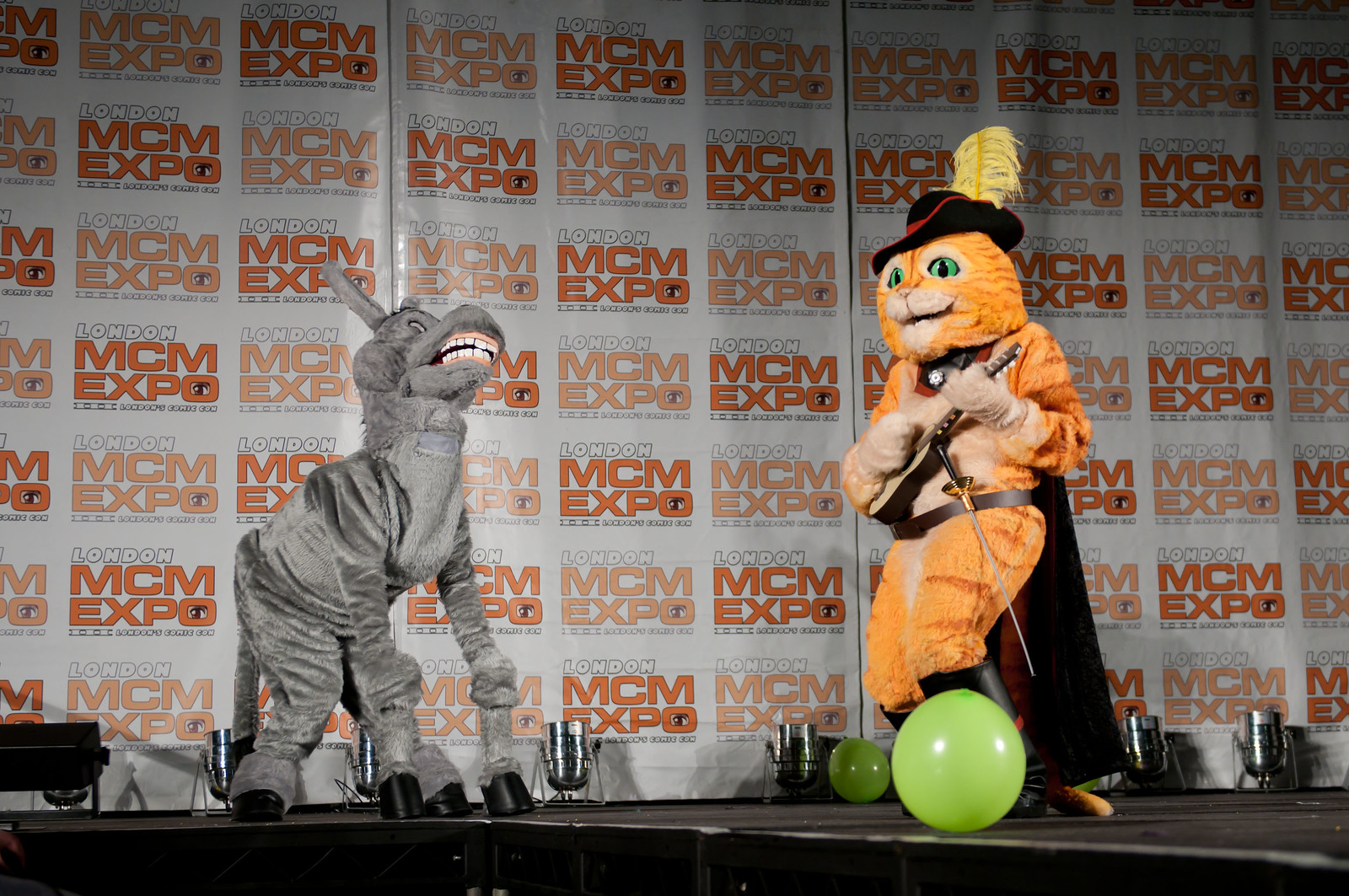In this vibrant photograph, two remarkably detailed costumed characters command the stage at the London MCM Expo. The imposing gray figure is a person donned in a frightfully realistic donkey costume, complete with elongated front limbs that mimic the animal's forelegs and menacingly exposed teeth beneath flared lips, evoking the beloved character from "Shrek." Beside him stands an equally striking representation of Puss in Boots, an orange cat character from the same movie, clad in a black cape, a black hat adorned with a yellow feather, and a small rapier sword at his side. The cat also skillfully plays a guitar, adding a lively touch to the scene. The stage itself is black and decorated with green balloons, enhancing the festive atmosphere. The backdrop features a gray wall with orange letters spelling "MCM Expo" and white letters below proclaiming "London," unmistakably anchoring this performance as part of the celebrated event.